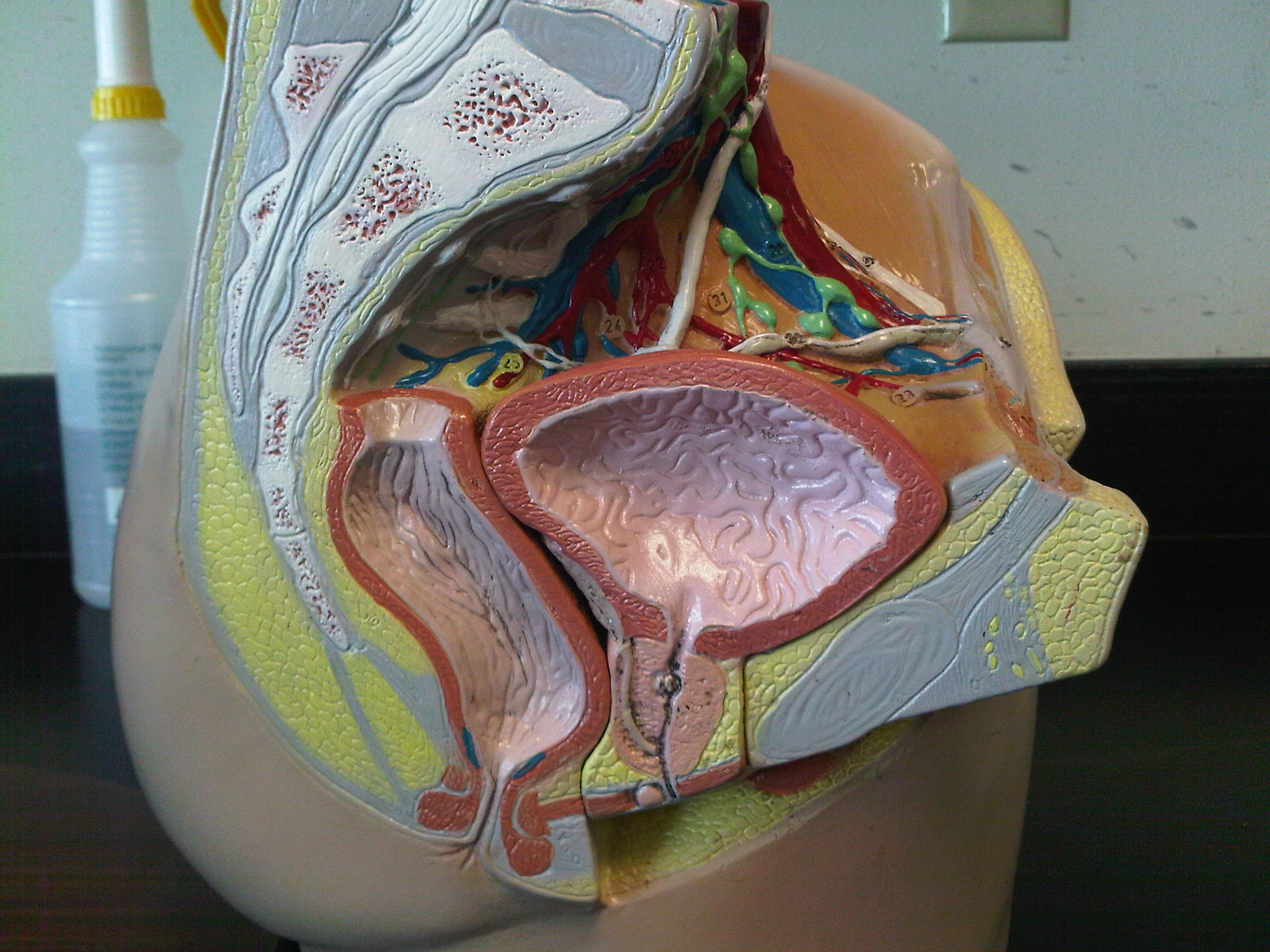The image depicts a detailed side-view anatomical teaching model set against a black countertop. The model illustrates various organ systems and layers within the body, highlighted in different colors. The model prominently features what appears to be the shape of the buttock and tailbone area, including a visible cutaway of the spine on the upper left. Organs such as the bladder and colon are distinctly shown, with the colon colored pink to represent the prostate area. Intricate networks of red, green, and blue veins and arteries are connected throughout the model, depicting the circulatory and lymphatic systems. The model is further detailed with yellow sections to indicate fatty tissues. Surrounding the anatomical display, a tall, clear spray bottle with a white and yellow trigger is partially filled with liquid, positioned to the left side of the image. Behind the model, a white wall serves as a neutral backdrop, with a partially visible wall plate at the top of the picture.